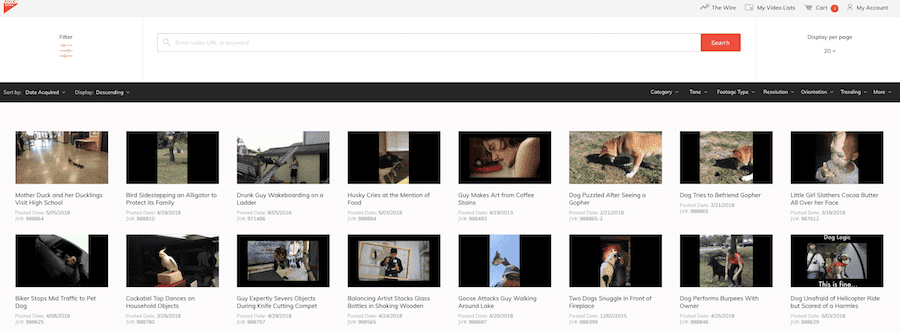The image is a horizontally oriented rectangular screenshot featuring a predominantly white background with black elements. At the top, there is a blank search bar. Below that, a prominent black navigation bar offers various clickable options. Underneath the navigation bar, a grid of small rectangular thumbnails, arranged in two rows with eight thumbnails per row, resembles miniature TV screens. Each thumbnail appears to represent a clickable video, reminiscent of YouTube video previews.

The upper-left thumbnail displays an image of a duck followed by its ducklings, accompanied by the caption, "Mother duck and her ducklings visit high school," along with a post date. Another thumbnail in the same row shows a dog staring at the ground with the text, "Dog puzzled after seeing a gopher." In the upper-right corner, there's an image of a baby with cocoa butter smeared on their face, captioned, "Little girl slathers cocoa butter all over her face." These thumbnails collectively suggest a collection of short, cute videos available for viewing.